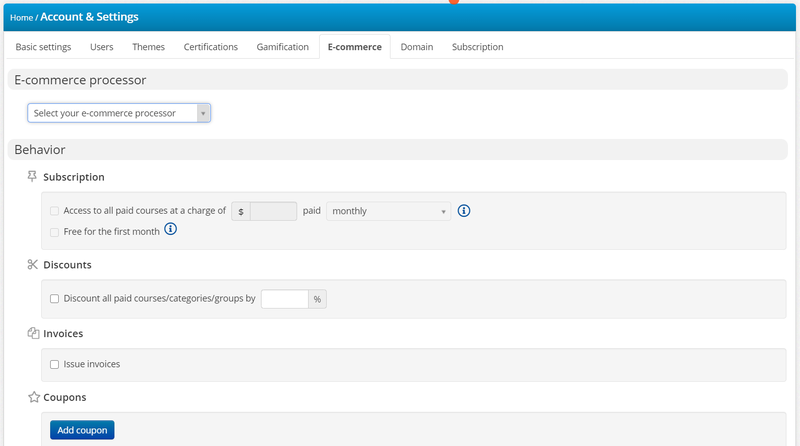The image appears to be a screenshot from a computer, specifically from an online settings or management platform. At the very top, there is a blue border. On the left side, there is a breadcrumb trail indicating "Home / Account and Settings."

Below the blue border, there is a row of white headings from left to right: "Basic Settings," "Users," "Themes," "Certifications," "Gamification," "E-commerce," "Domain," and "Subscription." The "E-commerce" tab is currently selected.

Underneath the headings, there is a gray border labeled "E-commerce Processor." Beneath this, there's a drop-down menu labeled "Select your E-commerce Processor."

Further down, there's a section titled "Behavior" with a "Subscription" subheading and a push pin icon next to it. A gray rectangle below contains the text: "Access to all paid courses at a charge of," followed by a bar and a drop-down menu set to "Monthly." It also mentions, "Free for the first month."

The next section is "Discounts," marked by a pair of scissors icon. It includes a gray area stating, "Discount all paid courses/category/groups by," with an empty field to input a percentage.

Following this, the "Invoices" section is denoted by an icon resembling paper. It offers an option labeled "Issue Invoices."

Lastly, there is a "Coupons" section with a star icon next to it and a blue "Add Coupon" button.